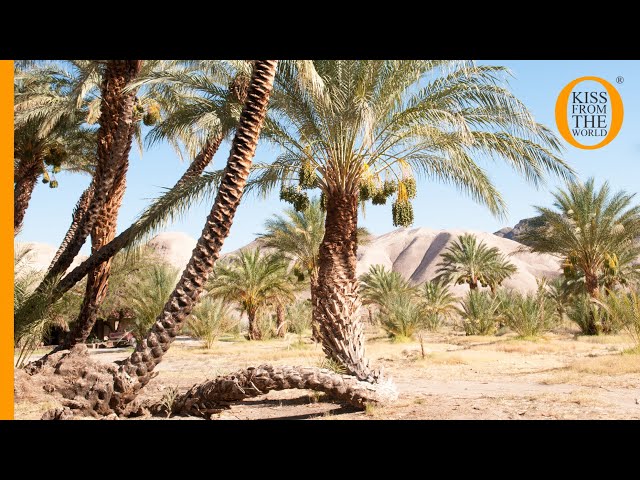This is a rectangular photograph featuring a serene, desert oasis landscape framed by thick black horizontal bars on the top and bottom, and a thin orange vertical border on the left side. The right side has no border. In the upper right corner, there's an orange circle with a transparent center encircling black text that reads "Kiss from the World." The scene itself showcases multiple healthy palm trees, some bearing indistinguishable green fruits, scattered across a sandy terrain. The sand is a yellowish hue, punctuated by undulating whitish sand dunes in the distance. The backdrop features a clear, cloudless light blue sky. Notably, a fallen palm tree with a visible curved trunk appears to be partially buried in the ground, adding a sense of timelessness to the tranquil desert setting.